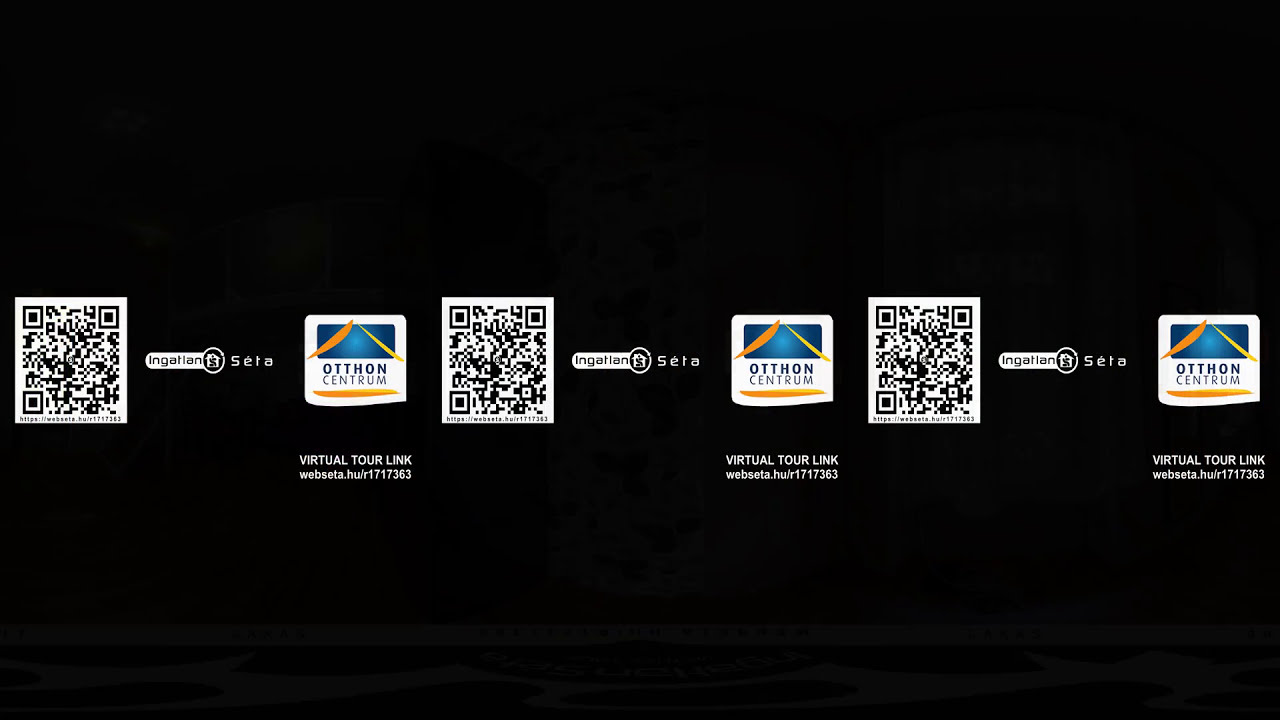This promotional image features a black background adorned with repeating QR codes and various brand logos arranged horizontally. On the far left, a QR code is positioned next to text that reads "Ingation F3 Cera" or "Ingation Seta," accompanied by a house-like logo that includes a money symbol. Adjacent to this text is another logo labeled "Othon Centrum," which displays a design incorporating two leaves, diagonal yellow and orange lines, and a blue rectangle in the center. Below these elements, the caption "Virtual Tour Link" is prominently displayed, along with the URL "MEBSETA.HUR1717383." These elements repeat in a banner-like format across the image, underscoring its purpose as a promotion for a virtual tour link. The text and design elements seem to be in a foreign language, enhancing the sophisticated and international appeal of the promotional content.